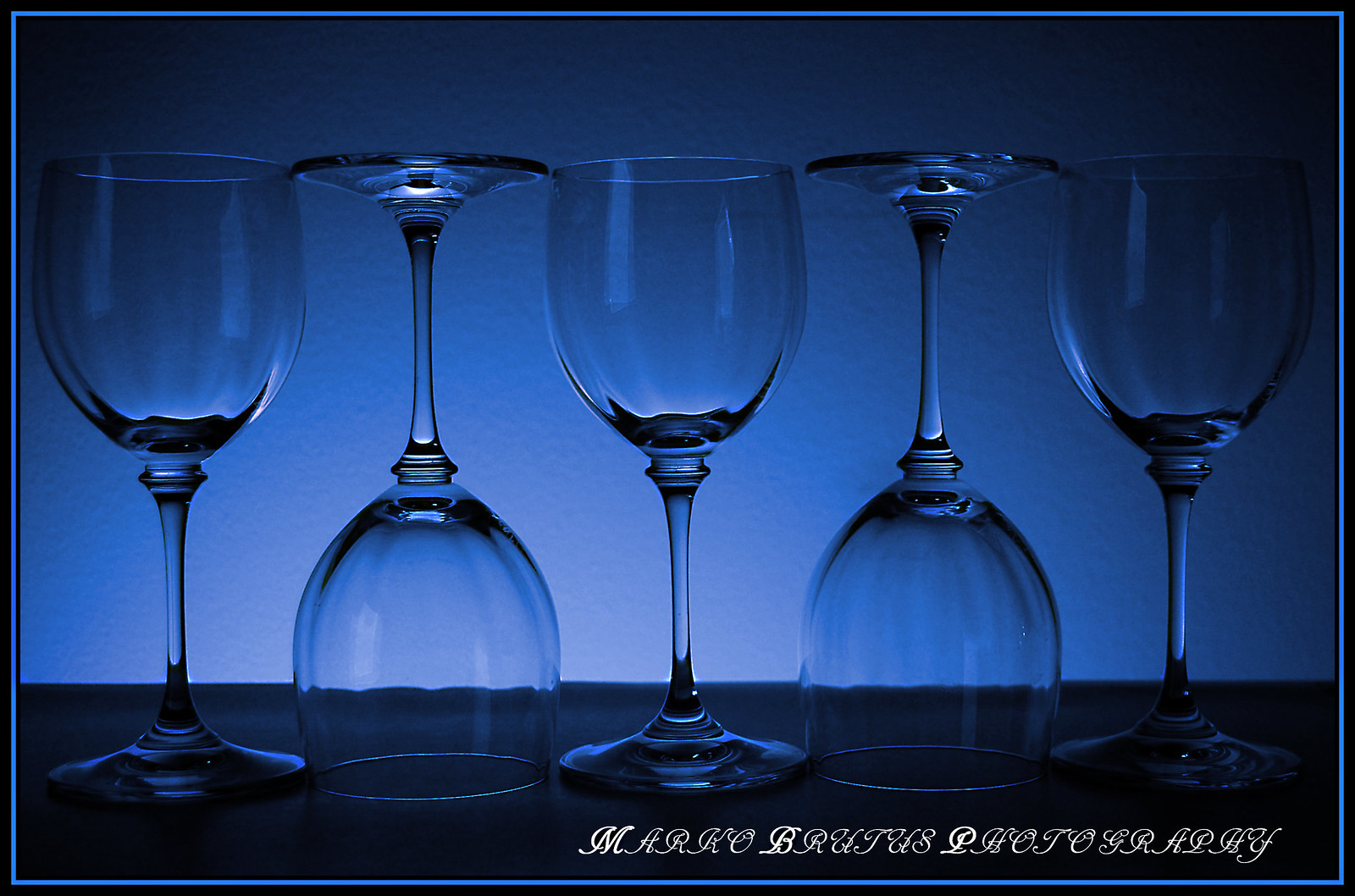The photograph, set against a blue-hued background, features a professional arrangement by Marco Brutus Photography, as noted in stylish cursive at the bottom right. The image showcases five elegant, empty wine glasses with a circular base and thin stem that tapers upwards into a traditional wine glass bowl. Their arrangement alternates in orientation: the first, third, and fifth glasses stand upright, while the second and fourth are flipped upside down. This artistic composition reveals a pattern that stretches across the entire width of the image and occupies most of its height. A dark surface supports the glasses, contrasting subtly with their translucent form. The background displays a gradient effect, with a brighter center light source fading into darker shades towards the edges. This lighting creates reflections on the stems and bowls of the wine glasses, adding depth and dimension. The photograph is encased in a thin blue border, enhancing its visual appeal, and exudes a sophisticated, artistic ambiance.